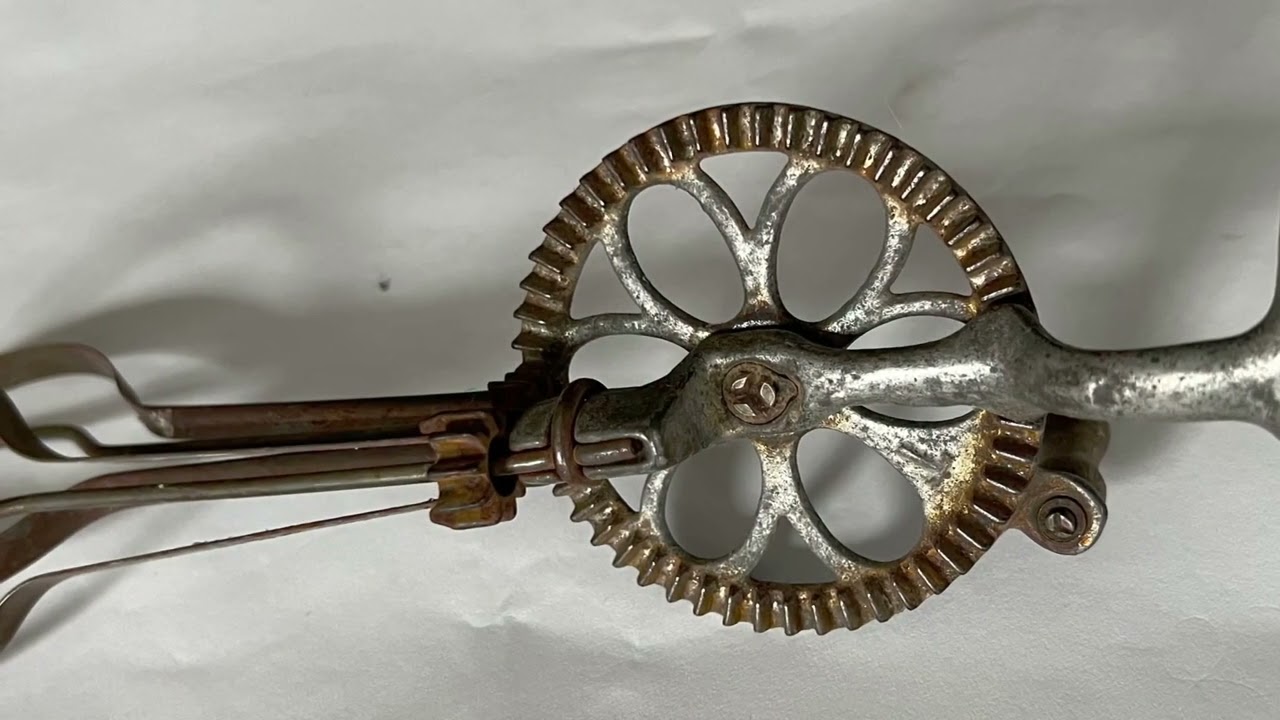This is a highly detailed close-up photograph of an old, rusted metal tool, possibly an antique egg beater. The image focuses on the central mechanism, featuring a large, stainless steel wheel with evenly spaced etched lines around its circumference. Within this wheel, six small circles are arranged in a flower-like pattern. Extending across the front of the wheel is a long, slender piece of metal that protrudes from both sides, held firmly in place by a bolt at the center of the wheel. The tool lies on its side against a white background, most likely butcher paper, which shows indents from the tool. The overall patina and rust on the metal indicate significant age and wear. The detailed gear system and teeth suggest it's designed for smooth rotational movement, typical of an egg beater's crank mechanism, although the picture is too zoomed-in to confirm the entire structure or handle. This could potentially be an eBay listing shot, but no additional context or pricing information is provided.